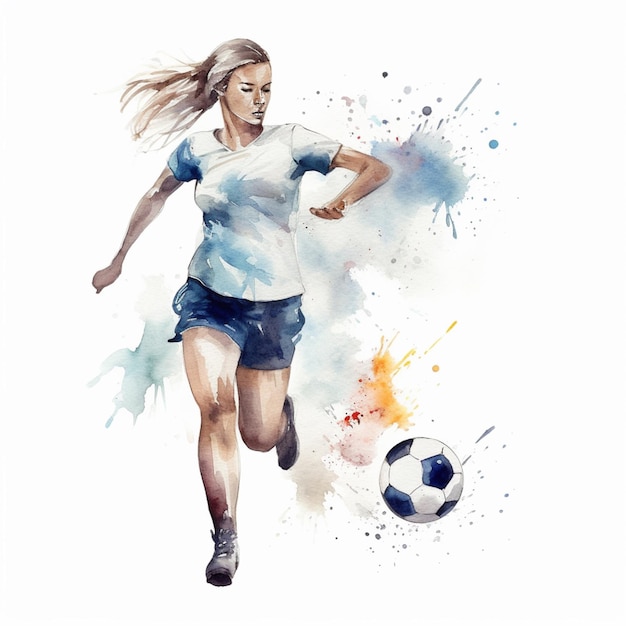The image is an illustrated, watercolor depiction of a female soccer player in mid-action. She has long, flowing blondish-brown hair and is wearing a white t-shirt with blue tie-dyed-like splashes and dark blue shorts. On her feet are black and white running shoes or cleats. Her stance suggests she is either chasing or preparing to kick a soccer ball positioned to the right of her, which is accompanied by splatters of mud, orange, and red paints, adding a dynamic sense of movement and energy to the scene. The splashes also extend around her right leg and foot, giving an impression of injury or intense action. The background features additional splashes of blue, gold, and rose-colored paint, creating an explosive, vibrant backdrop that contrasts with her focused demeanor. The intricate details of the splatters and colors on both her shirt and the surroundings enhance the sense of motion and drama, prompting intrigue about the unfolding story within the illustration.